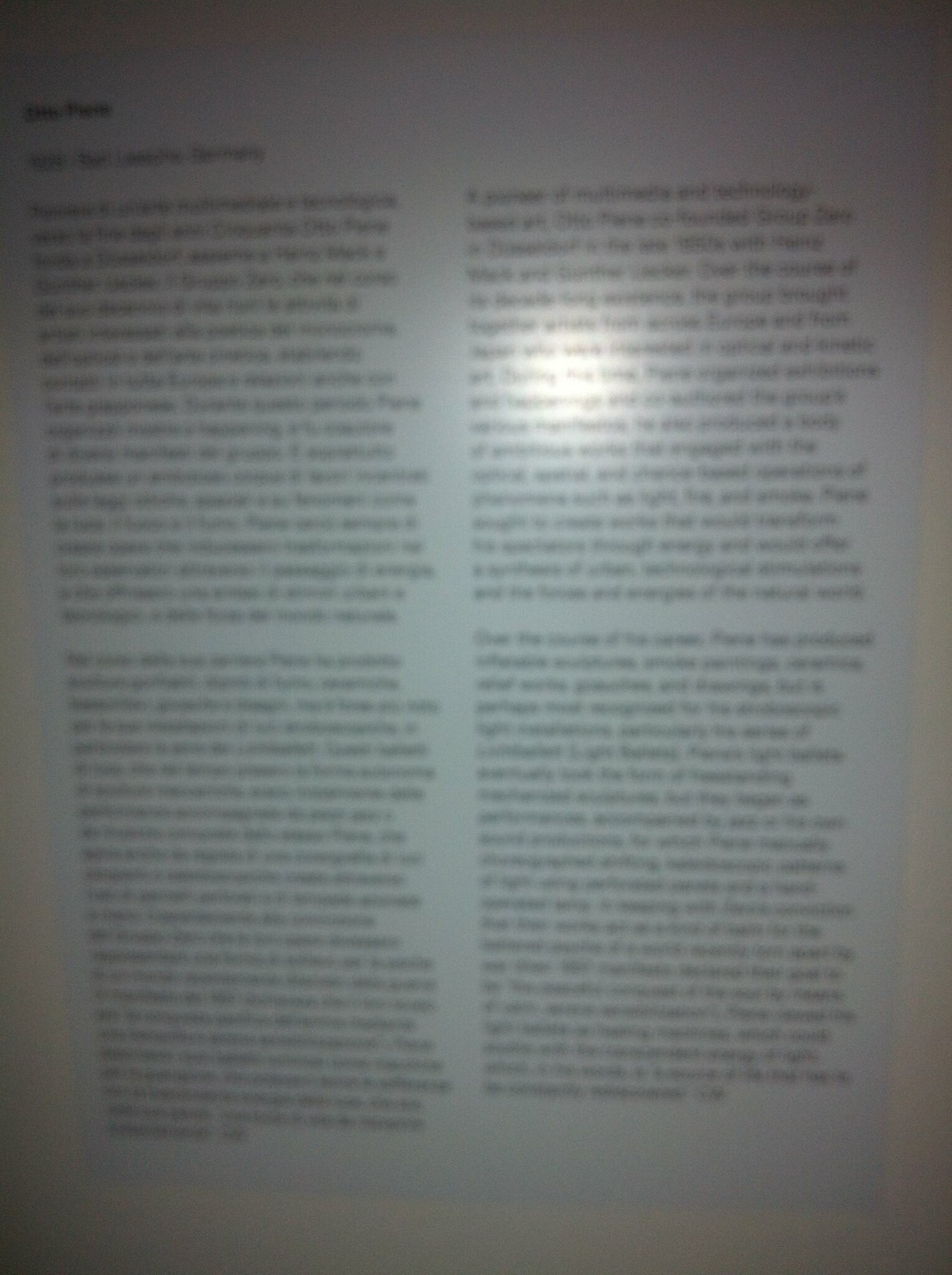This close-up photograph depicts a very blurry page taken from a book, making the text unreadable. The page is divided into four evenly-sized sections of text, with each column comprising two paragraphs. In the upper left corner, there is a boldfaced title, and just below it, a subtitle can be discerned. The alignment of the text is flush on the left, creating a neat left margin, while the right edges are uneven. A bright, white glare from a light source is visible above the center of the page, particularly in the upper right quadrant of the text. The page rests on a white surface, blending with its own color, further emphasizing the indistinctness caused by low lighting conditions.